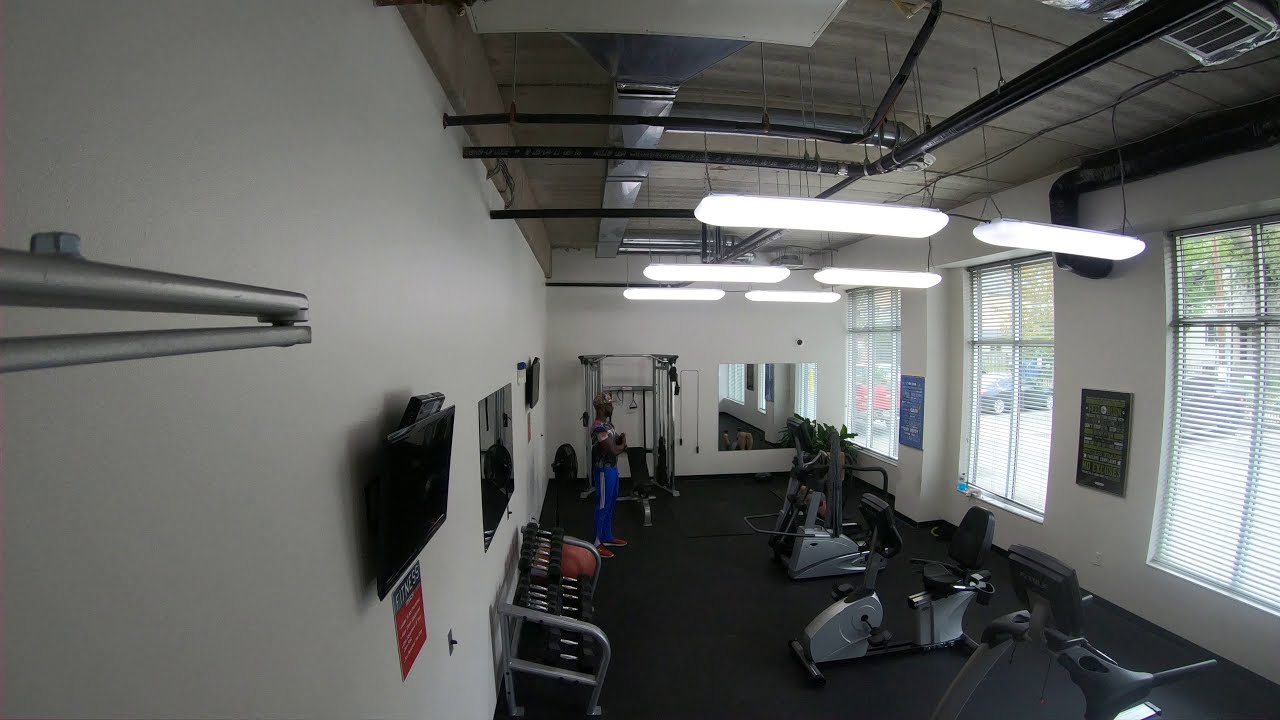The photograph captures the interior of a small gym, possibly connected to a workplace, characterized by its clean, modern look with off-white, cream-colored walls. Overhead, rectangular fluorescent lights with rounded corners illuminate the space, while black air conditioning pipes run along the ceiling. In the center-left of the image, an African American man with dark brown skin, wearing a black short-sleeve shirt, deep ocean blue sweatpants, red tennis shoes, and a hat stands with his hands crossed, facing the center of the room. The gym is equipped with various cardio machines, including a stationary bike, an incline machine, and a treadmill toward the back. To the forefront, there's a shelf holding black dumbbells, made of metal bars. A flat-screen TV is mounted on the left wall, though it's turned off. In the background, large mirrors and several windows let in daylight, offering a view of the outside parking lot. The room is devoid of other people, suggesting a quiet, perhaps early hour in the day. On the walls, which are largely undecorated, plaques and picture frames hint at recognition or decor that’s not legible from this distance.